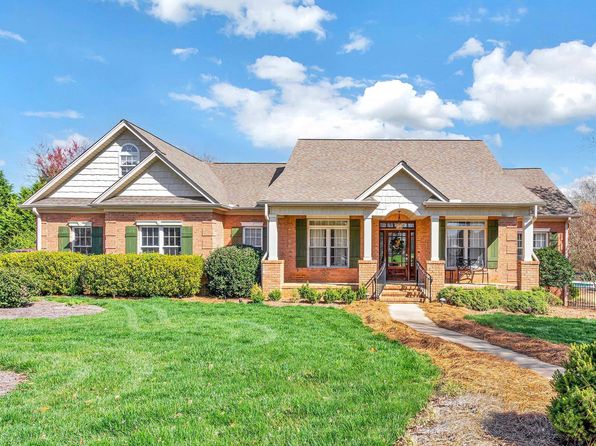The image showcases a private home with a green front yard bordered by patches of yellow grass. The house is predominantly made of light-colored bricks and features white siding on the upper section, topped with a tan-colored roof. Green shutters adorn the several visible windows, adding a touch of color to the front facade. The house appears mainly as a single-story structure with a second story visible on the left side, highlighted by a window and a slanted roof. The front yard includes various bushes and hedges, with taller bushes on the left side compared to the right. A clear blue sky with light clouds forms the backdrop. A central pathway, flanked by small patches of yellowish grass, leads to a small staircase with three or four steps that ascends to the front door. The yard also features lush green grass and several trees situated at the left and right corners of the image.